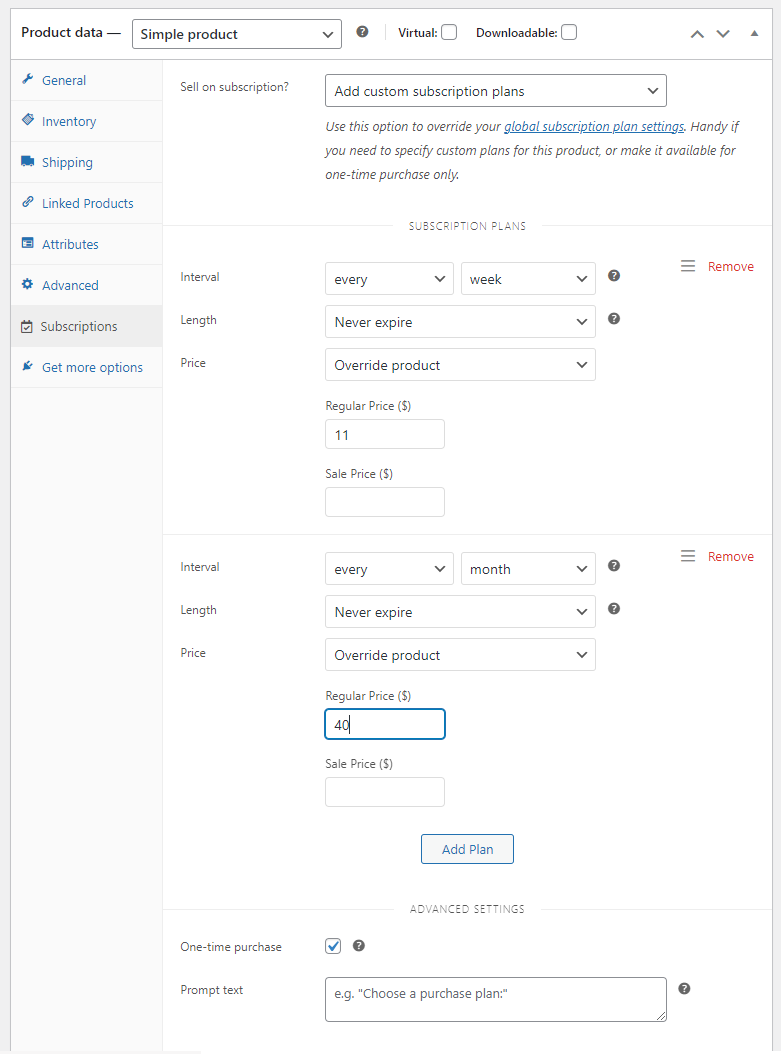This image is a detailed view of a subscription plan creation page within an admin panel. At the very top left corner, "Product Data" is visibly written in small black letters. Adjacent to this text is a drop-down box currently set to "Simple Product," followed by two unchecked check boxes labeled "Virtual" and "Downloadable."

On the left side, a grey vertical panel extends from the top to the bottom of the page, listing several categories each accompanied by an icon. These categories include "General," "Inventory," "Shipping," "Linked Products," "Attributes," "Advanced," and "Subscriptions," with "Subscriptions" highlighted in dark grey, indicating it is the selected category.

Occupying the entire right side of the page are the settings for subscription plans. At the top left, the section is titled "Set on Subscription," alongside a drop-down box set to "Add Custom Subscription Plans." Directly below, the section for specifying intervals is presented, featuring two drop-down boxes: the first is labeled "Every" and the second is set to "Week," indicating a weekly subscription interval.

Below this is a section for pricing details. It lists "Regular Price," set at $11 for the weekly subscription. There is another section that defines a different interval: the drop-down boxes here set the interval to "Every Month," with the length specified as "Never Expire." The "Regular Price" for this monthly subscription plan is marked at $40.

In the center below these settings, there is a button labeled “Add Plan,” presumably for adding these subscription plans to the product.